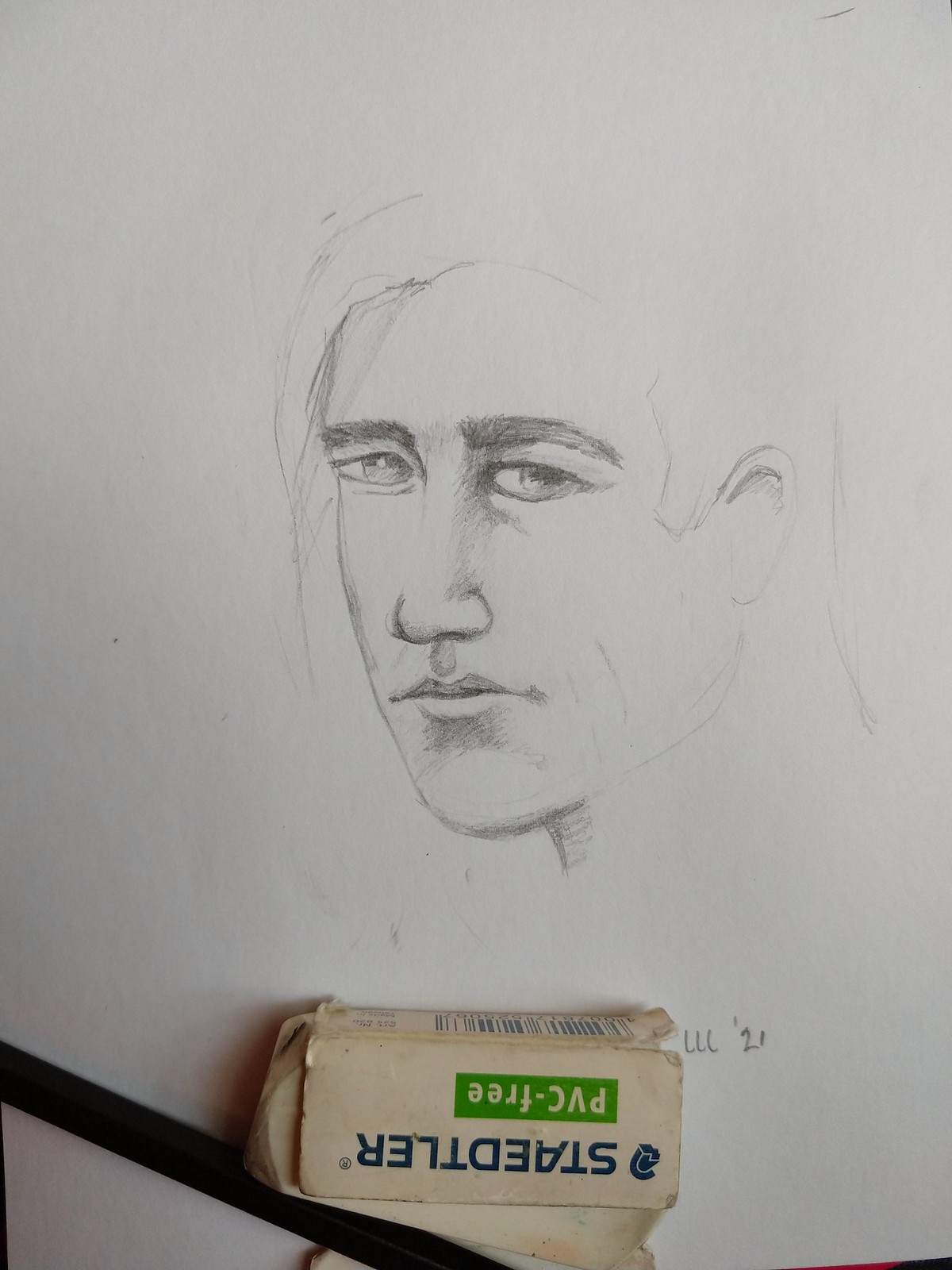This image, set against a light orchid-colored piece of paper, features a detailed pencil sketch of a young man. His hairstyle is asymmetric, with short hair visible over one ear and longer strands sweeping across his face, reaching down to his cheek on the other side. The young man has prominent, heavy eyebrows and large, melancholic eyes that add a depth of emotion to the portrait. At the bottom of the image, there is a rectangular package marked with the brand name "Staedtler" in bold blue letters. Additionally, a green square on the package displays "PVC free" in white text. Lying across the bottom of the package is a slender black rod, possibly a pencil or an artist's tool, adding a practical touch to the artistic scene.